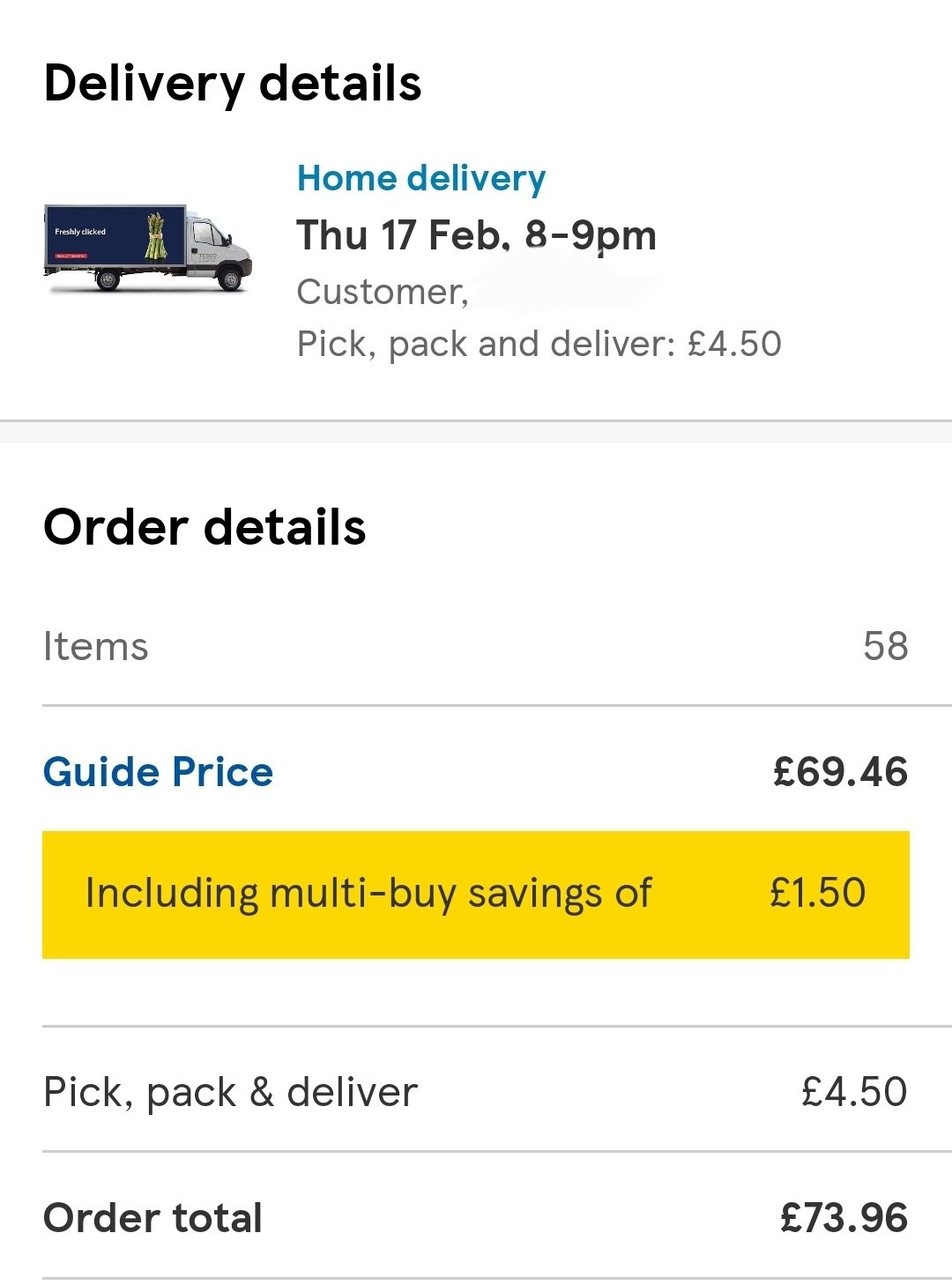The screenshot displays detailed delivery information for a package, likely from a British home delivery service. Dominating the upper portion is a digitally-rendered image of a white delivery truck with "Freshly Clicked" emblazoned in bold on its blue side panel. Notably, a bundle of asparagus, tied off with rubber bands, is stacked vertically at the edge of the truck, lending a fresh and organic touch to the visual.

Below the truck, the delivery details are prominently outlined:

- **Delivery Details**
    - **Home Delivery**: Thursday, 17th of February, 8 to 9 p.m.
    - **Customer**: Pick, pack, and deliver
    - **Charge**: £4.50

A grey line demarcates this section from the order summary below, which provides a meticulous breakdown:

- **Order Details**
    - **Items**: 58
    - **Guide Price**: £69.46 (includes multi-buy savings of £1.50)

Following another grey separator line, the delivery charge is reiterated:

- **Pick, Pack, and Deliver**: £4.50

This brings the **Order Total** to £73.96, emphasized in bold text. The background remains plain white, ensuring all text and figures are sharp and clear. The image's overall design is clean and structured, with thin grey lines and a yellow highlight used to segregate different sections.